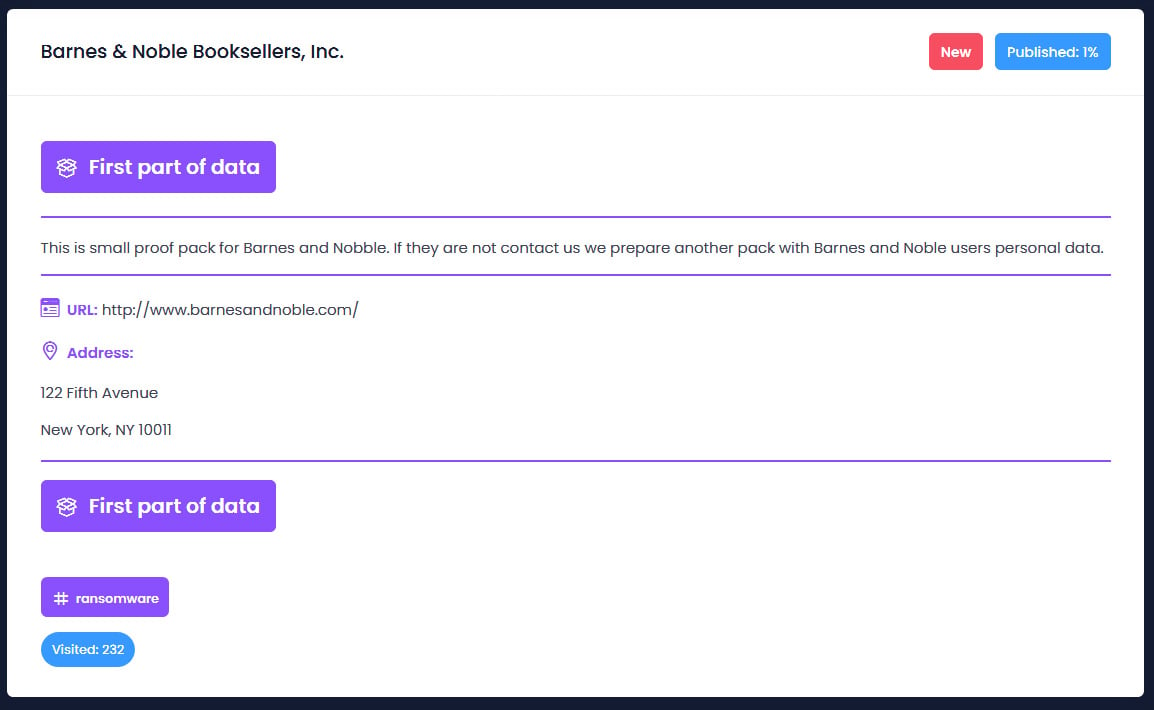A detailed and cleaned-up caption for the image screenshot could be:

---

The image is a screenshot on a white background featuring a message from Barnes & Noble Booksellers, Inc. It contains a prominent red rectangle with the words "new" and "published" highlighted in white. Adjacent to this is a blue rectangle with "1%" written in white text. The screenshot includes a purple rectangle that appears to hold the first part of the data. This is a small proof pack intended for Barnes & Noble. The message warns, "If they are not, contact us. We prepare another pack with Barnes & Noble users' personal data." Additionally, the image features a URL: "www.barnesandnoble.com," and a physical address: 122 5th Avenue, New York, New York, 10011. Another purple rectangle is present, listing further data, and there are repeated mentions of a pound sign followed by "Ransomware." A blue oval is also notable in the screenshot, stating "visited: 232."

---

This caption is descriptive, structured, and free from grammatical issues, providing a clear understanding of the image content.